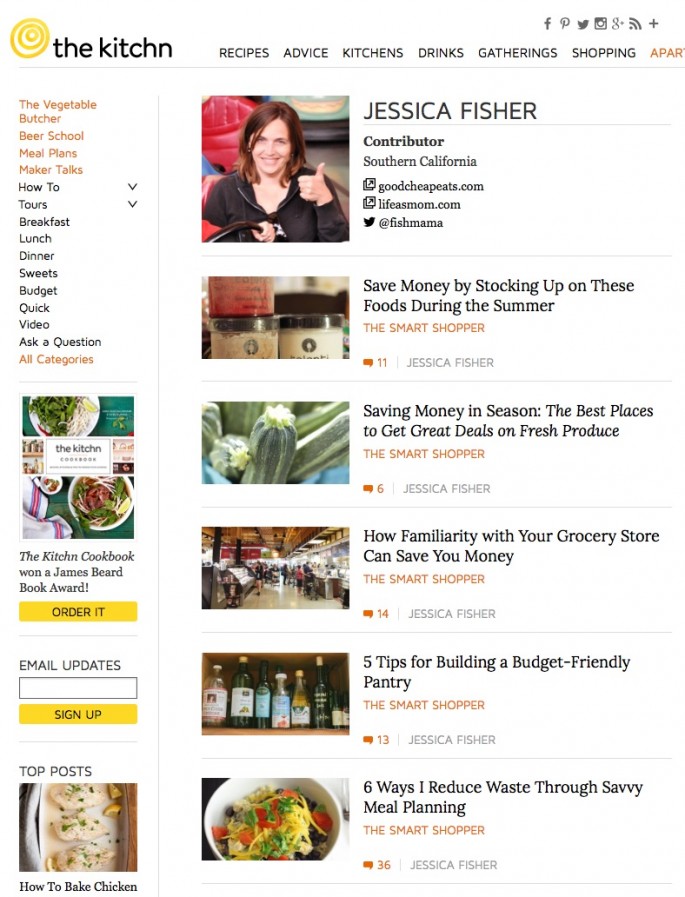The webpage from the kitchen-themed site features a plethora of images arranged together, establishing a visually engaging layout. Dominating the page is a highly visible section that promotes the option to order a cookbook. There's also a subscription form prompting users to sign up for email updates by submitting their email addresses.

A featured top post guides readers on "How to Bake Chicken," complemented by various highlighted articles. One article discusses Southern California resident Jessica Fisher’s strategies to save money by stocking up on specific foods during the summer. The "Smart Shopper" series provides valuable tips including: "Saving Money in Season: The Best Places to Get Great Deals on Fresh Produce," "How Familiarity with Your Grocery Store Can Save You Money," "Five Tips for Building a Budget-Friendly Pantry," and "Six Ways I Reduce Waste Through Savvy Meal Planning." Each piece in the series focuses on economical and sustainable shopping and meal planning practices.